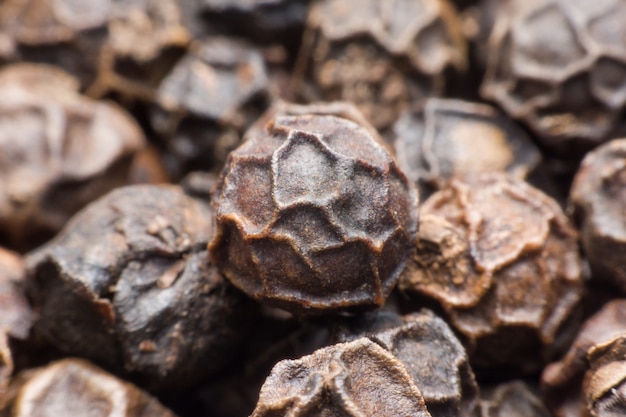This close-up color photograph captures a large clump of small, round, dark brown objects that appear distinctly biological in origin, resembling seeds or dried nuts. The vertical rectangular image presents a top-down perspective with approximately 15 to 20 of these objects in frame, all clumped together. The primary focus is on one object at the center of the image, which is sharply in focus, while the others fade into a soft focus in the background. This central object features a raised, veiny pattern of indented, imperfect circles that curve and intersect all over its surface, giving it a textured appearance. The collective resemblance to something natural and uniform, yet individually unique, adds a layer of curiosity, making them look like potential seeds or dried fruits with intricate surface details.